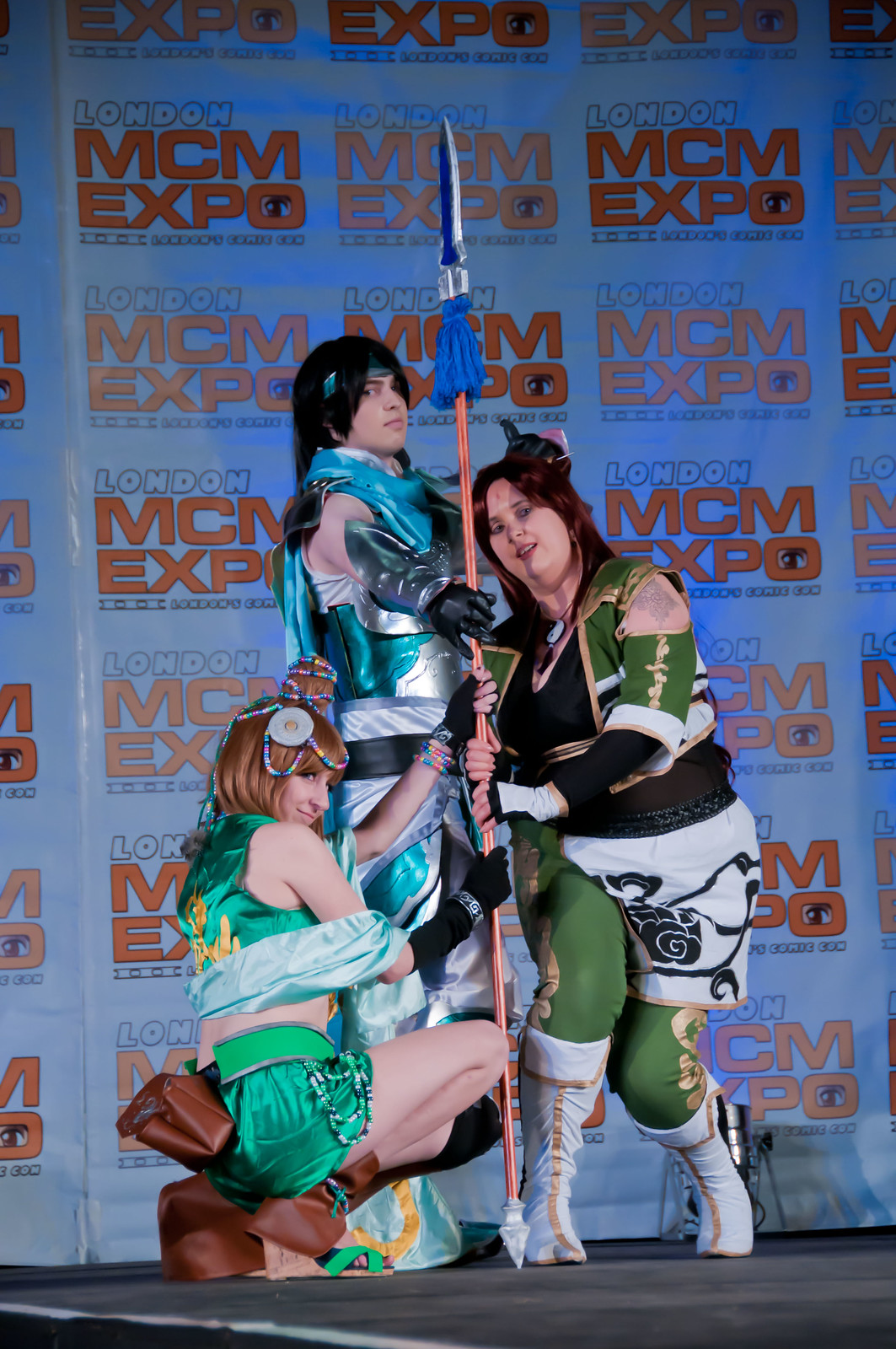The photograph taken at the London MCM Expo captures a vibrant cosplay scene on stage, featuring three characters wielding a tall jousting spear with a blue blade and a brown pole capped in silver. The backdrop displays "London MCM Expo" in distinct lettering, with "MCM Expo" in bold red font and "London" outlined in blue. 

To the left, a woman with long red hair, intricately styled with beads and shaped into a cone, is slightly kneeling. She is dressed in a green skirt and top, complemented by brown leg coverings. 

In the center, a man with long black hair stands, adorned in an aqua and silver suit that includes a cape, a headband, black gloves, and silver arm accessories. 

On the right, another woman, with pink blonde hair, is crouching. She is clad in white boots, green pants, and a striking black and white dress featuring green shoulders and arm sleeves.

Each cosplayer's costume is detailed and colorful, speaking to the effort and creativity that characterize the vibrant atmosphere of the expo.